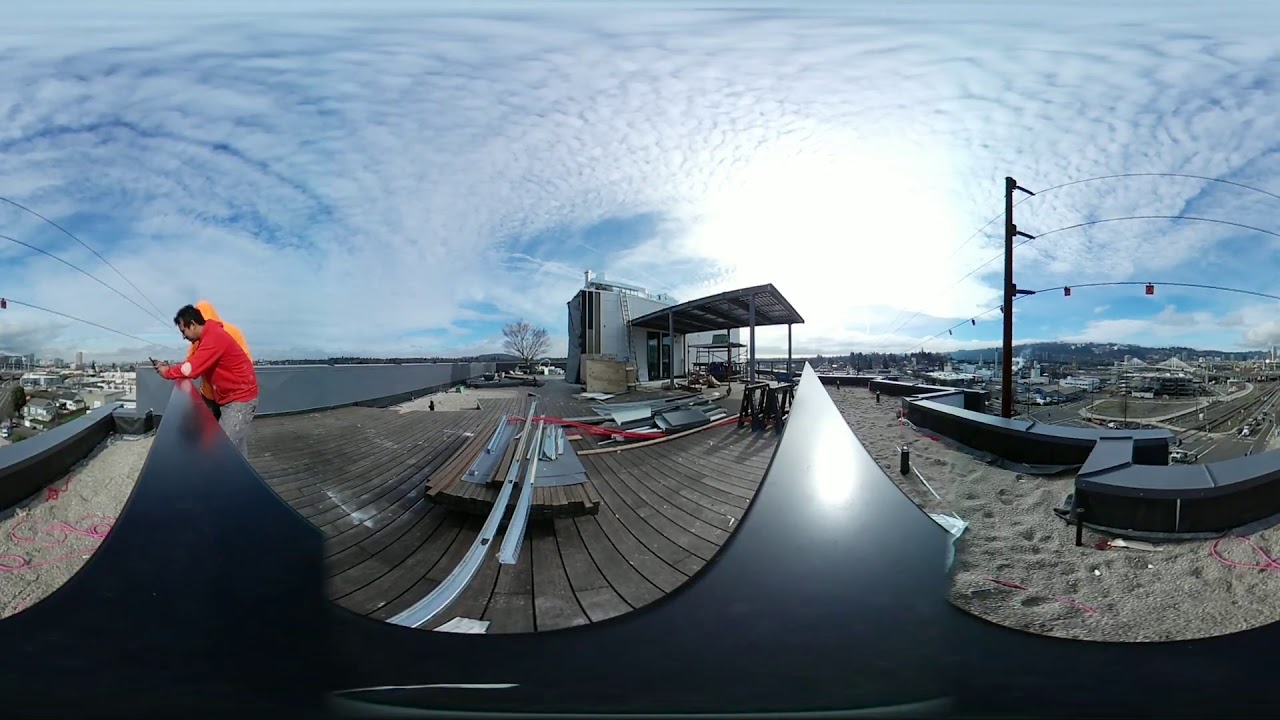This panoramic photograph, taken outdoors during the day, showcases a high rooftop scene with a fisheye lens effect that visually distorts the image, making it appear rounded. The sky, filled with white clouds and streaks of blue, covers the top half of the image. To the left, two men lean on a black metal railing that runs along the rooftop's edge; the man in front wears a red sweatshirt and holds a cell phone, while the man behind him, harder to see, wears an orange hoodie. They're positioned near the edge, possibly looking down at a lower tier covered with sand.

In the center of the photograph, construction work is evident with wooden planks being installed vertically and debris scattered around. A small, square stone building with a long archway stands out, potentially serving as the entrance to the rooftop. Further to the right, the fisheye effect causes power lines to appear as if they are arcing above the scene. Here, additional construction materials such as scaffolding, a ladder, and sashes are visible against a light blue or gray building with a flat awning. The background reveals a distant cityscape on both sides of the image and, towards the water at the edge, suggesting a location near a pier or an urban waterfront.